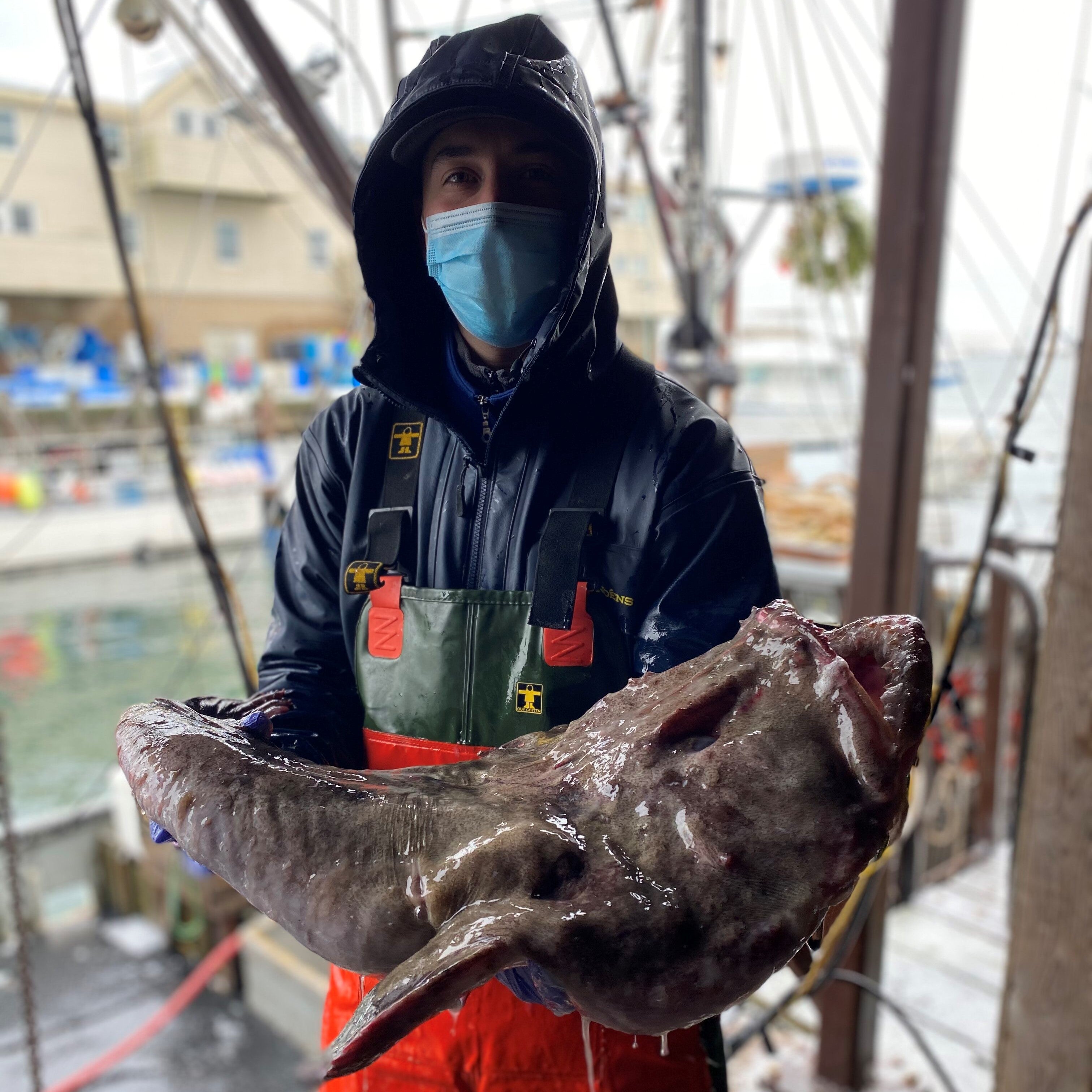In this image, a fisherman, outfitted in a navy blue coat and a green and red apron over heavy-duty gear, stands prominently in the foreground, holding a large, ungainly, and somewhat reflective grey fish. The fisherman is masked, adding to the sense of preparedness against the elements. The fish, possibly a monkfish, has a decidedly unattractive appearance, with its muddy coloring and somewhat iridescent sheen. Behind the fisherman, the scene transitions into a blurred background featuring an assortment of fishing boats, a busy pier, and port buildings, including a noticeable three-story warehouse. The colors in the image range widely from bright orange, dark forest green, various blues, to earthy tones like beige, tan, and brown. The sky is fully overcast, suggesting a cloudy day with no visible sunlight, adding a muted atmosphere to the bustling maritime setting.